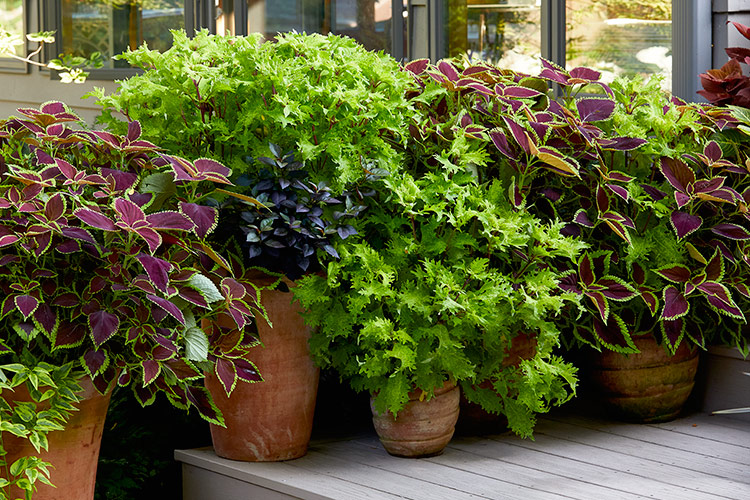This outdoor daytime photograph captures a detailed arrangement of potted plants in a garden area by a building with large glass windows in the background. The image, approximately five to six inches wide and four inches high, displays a variety of plants placed on a gray wooden platform and around it. Starting from the lower left corner, there's a red terracotta pot overflowing with two plants, including a small hosta with dark green and light green leaves. Above this, there's another hosta with larger spade-shaped leaves featuring red centers and light green edges. To the right, elevated on the wooden platform, another terracotta pot contains plants with striking dark bluish, purpley-black leaves. Moving further right, there are plants with curling leaves and another hosta with red and green coloration. On the far right, a burnt orange leaf emerges from the side. The background showcases windows reflecting greenery, adding depth and context to this vibrant garden scene.